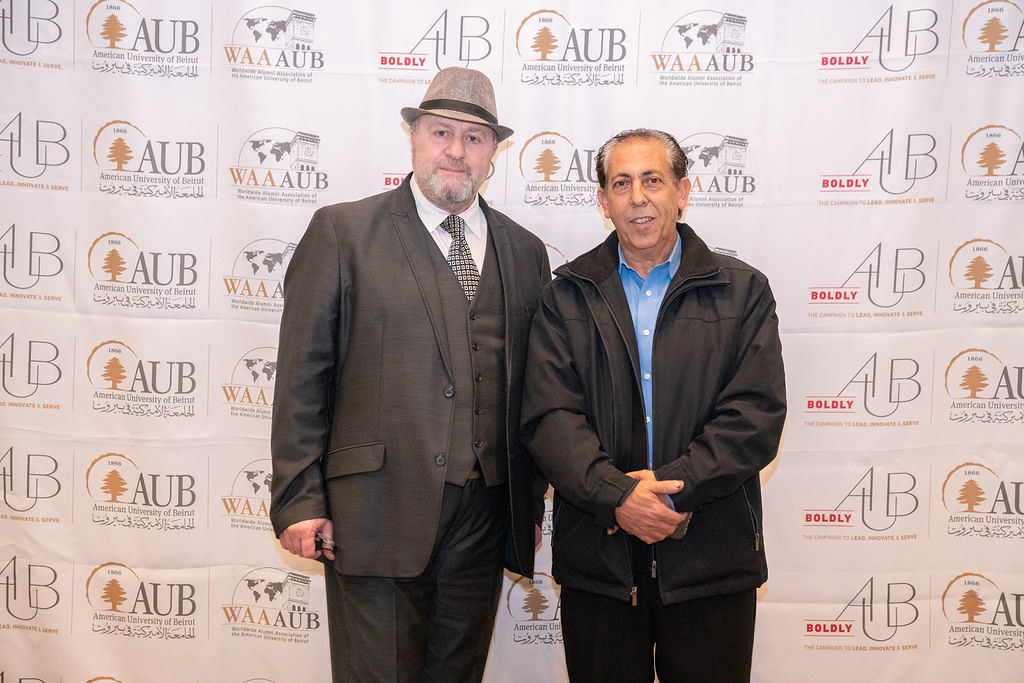The photo showcases two older gentlemen standing side by side in front of a banner from the American University of Beirut that prominently features the word "boldly" in red letters and "AUB" in black letters on a white background. The man on the left is wearing a distinctive ensemble that includes a brown suit with a tie, a matching tan and brown hat, and has a mustache and short beard. The man on the right is dressed in a black jacket over an open-collared blue shirt and dark pants. Both men appear to be smiling, exuding a sense of camaraderie and style.